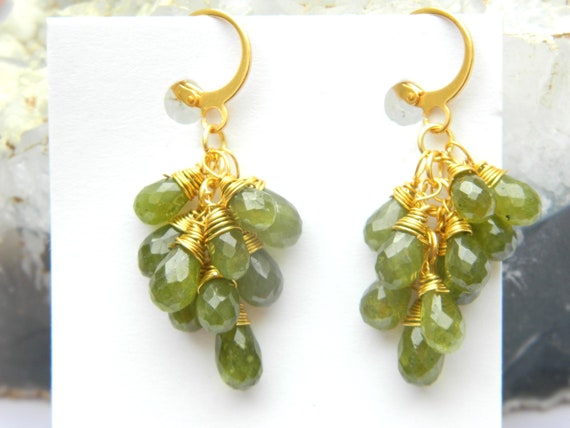This photograph features a pair of elegant earrings displayed on a small, square-shaped white paper card, which serves as a holder. The earrings hang from two circular holes punched at the top of the card. The background is blurry and gray, with indistinct shapes that don't distract from the focal point.

Each earring consists of several elements: at the top, golden circular loops attach the earrings to the card. Hanging from each loop are additional gold rings that connect to a cluster of approximately ten green glass or jade-like jewels. These jewels are teardrop-shaped, with faceted edges, resembling small light bulbs or grapes. The green jewels are meticulously secured at their bases with gold coils, creating a striking and sophisticated appearance. The green bulbs, which have a blue tint at their tops, dangle gracefully, forming a design reminiscent of grape clusters.